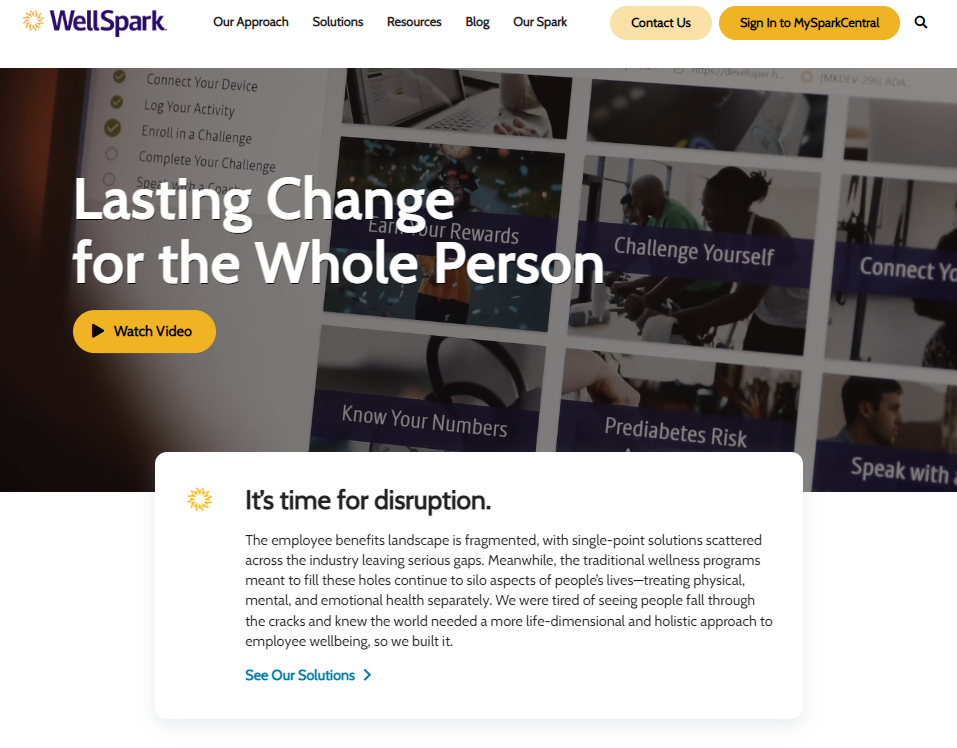The web page showcases a prominently designed, user-friendly interface. In the upper left corner, the logo of Wells Park is displayed, featuring a small, yellow sun-shaped circle followed by the words "Wells Park" in a bold, deep purple font. At the top of the page, a navigation bar provides access to various sections including "Our Approach," "Solutions," "Resources," "Blog," and "Our SPAC." 

Adjacent to these links, "Contact Us" is highlighted within a light cream-colored bubble, drawing users' attention. On the far right, an orange bubble contains the prompt "Sign in to My SPAC Center," encouraging users to log in.

Centrally located below the navigation bar is a large, eye-catching image displaying people engaged in various activities, reflecting the site's community-oriented focus. Superimposed on this image, large white text reads "Lasting Change for the Whole Person," with a yellow bubble below containing the call-to-action "Watch Video."